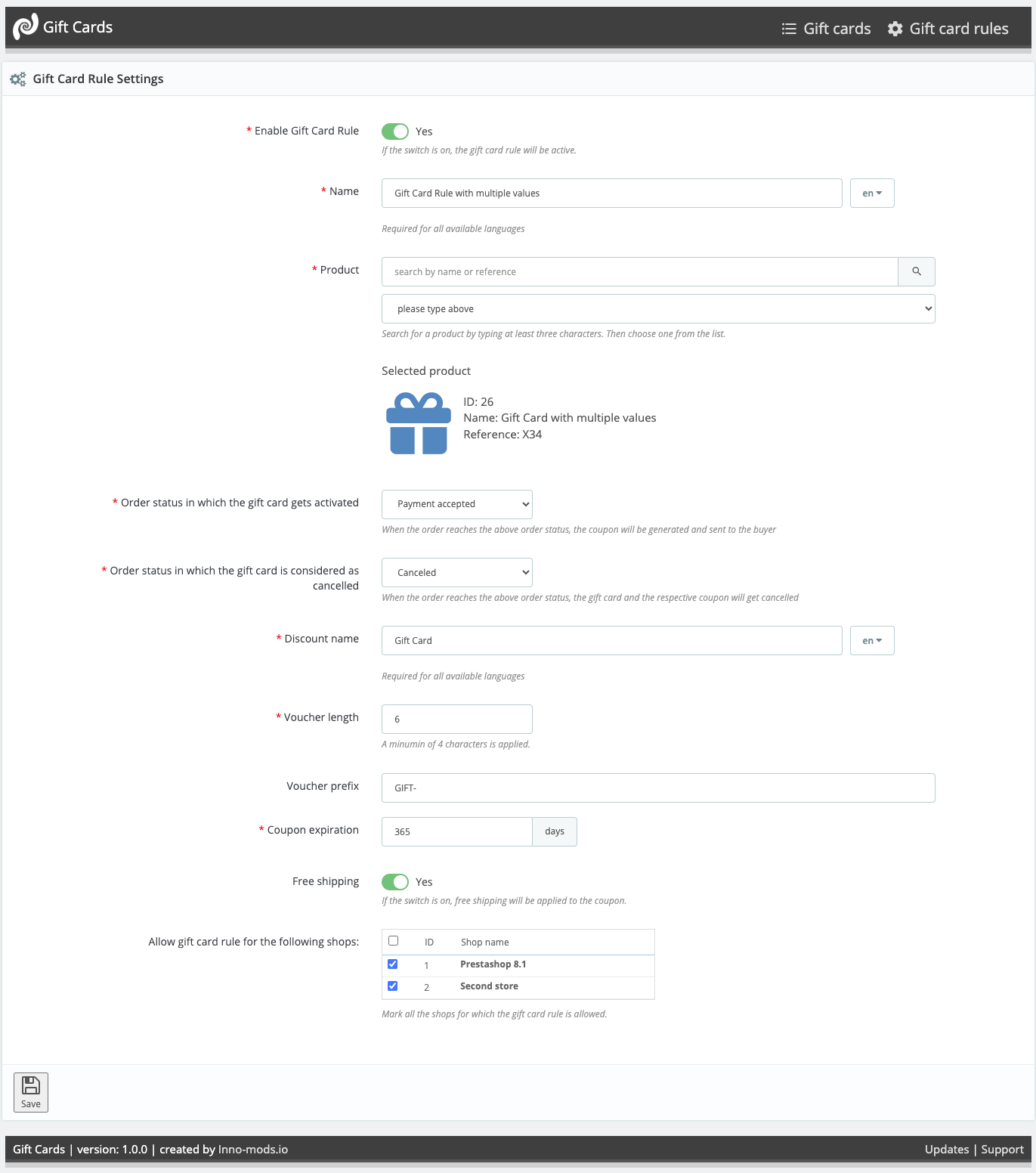***Gift Card User Interface Detailed Description***

The image showcases a gift card user interface (UI) with an elegant and functional design. Dominated by a black background, the UI features a prominent white swirl motif in the center which accompanies the text "Gift Cards." To the right of this is an interface element consisting of three dots followed by three horizontal lines. The text "Gift Cards" appears again in white, next to a gear icon indicating settings, followed by the text "Gift Card Rules."

Below this header section, the interface includes a circular icon with two satellite circles, labelled "Gift Card Rule Settings." The section highlights that the "Enable Gift Card Rule" option is toggled to "Yes" via a visible slider switch. A note clarifies that if the switch is on, the gift card rule will be active.

The description continues with a setting for the "Name" of the gift card rule, marked by a red asterisk indicating it's required. A dropdown menu displays "EN" for English, and an annotation specifies this is required for all available languages. Adjacent to this is a product search feature with a magnifying glass icon, instructing users to search by name or reference. It prompts users to type at least three characters to search for a product, and then choose from the resultant list.

Following the product search, there is a subsection labeled "Selected Product," featuring an image of a blue gift, described as Wedgwood blue. The product details listed include: ID 26, name "Gift Card with Multiple Values," and reference X34.

The interface further includes an order status dropdown, where "Payment Accepted" is selected. A note clarifies that when the order reaches this status, the coupon will be generated and sent to the buyer. There is also an order status to mark cancellation, where "Canceled" is selected. It specifies that the gift card and coupon will be canceled when the order reaches this status.

Additionally, the UI has a segment for the "Discount Name," again requiring input for all languages with "Gift Card" selected in English. Another setting, "Voucher Length," defaults to six characters with a minimum requirement of four characters. The voucher prefix is set as "gift-," and the coupon expiration is set to 365 days, meaning the coupon will expire in one year.

The feature for enabling free shipping indicates it is toggled to "Yes," which applies free shipping to the coupon. The UI also allows setting gift card rules for different shops, listing "ID Shop Name," with "PrestaShop 8.1" and "Second Store" both selected.

To the left of the interface, there is a Save icon for saving the configuration. At the bottom, a black bar displays the text "Gift Cards," flanked by a horizontal line, followed by "Version 1.0.0." Another line states "Created by inno-mods.io," and to the right, further options for "Updates" and "Support" are indicated by horizontal lines.